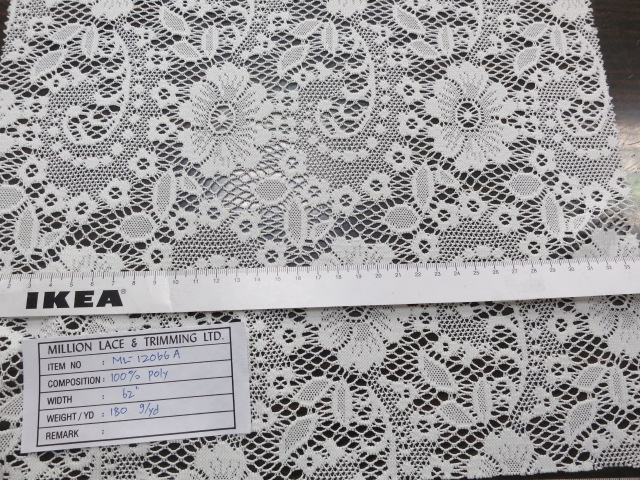This close-up photograph features a white lace fabric adorned with intricate flower and leaf patterns. The lace is positioned slightly skewed to the right, extending off the image on the bottom left and nearly reaching the bottom right. Dominating the center of the image is a white IKEA ruler marked with black numbers, which spans from the left to right edge, partially extending off both sides of the picture. Just below the ruler, on the left side, is an information card framed by a black-trimmed box. The card, titled "Million Lace and Trimming, LTD," provides essential details about the fabric: its item number, composition (100% polyester), width (62 inches), and weight (180 yards). Some of this information is handwritten next to printed labels, while the remarks section remains blank. The overall scene emphasizes the detailed inspection and presentation of the lace fabric's attributes.